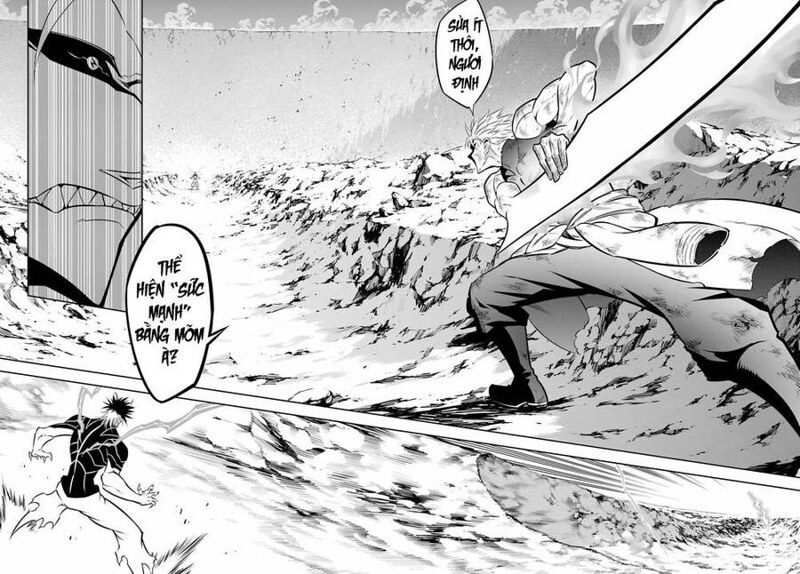This black-and-white manga comic page features intense, stylized artwork. The scene is divided into two primary panels, with speech bubbles in an unknown language, possibly Vietnamese. On the bottom left, there's a close-up of a small character with spiky hair, who has very black eyes with tiny white pupils, a grimacing expression, and spiked teeth. Vertical gray lines accentuate his visible anger. In the top right corner, a much larger figure dominates the panel. This character has spiky blonde hair, bulging muscles, and a shirt tied around his waist. He wields a partially-visible object, possibly a sword, gripping both the handle and the blade, and appears to be leaning it behind him. This large figure seems to be confronting another character in the distance, who is surrounded by electrical energy. The background features a textured, rocky landscape, adding to the tense atmosphere of the scene.